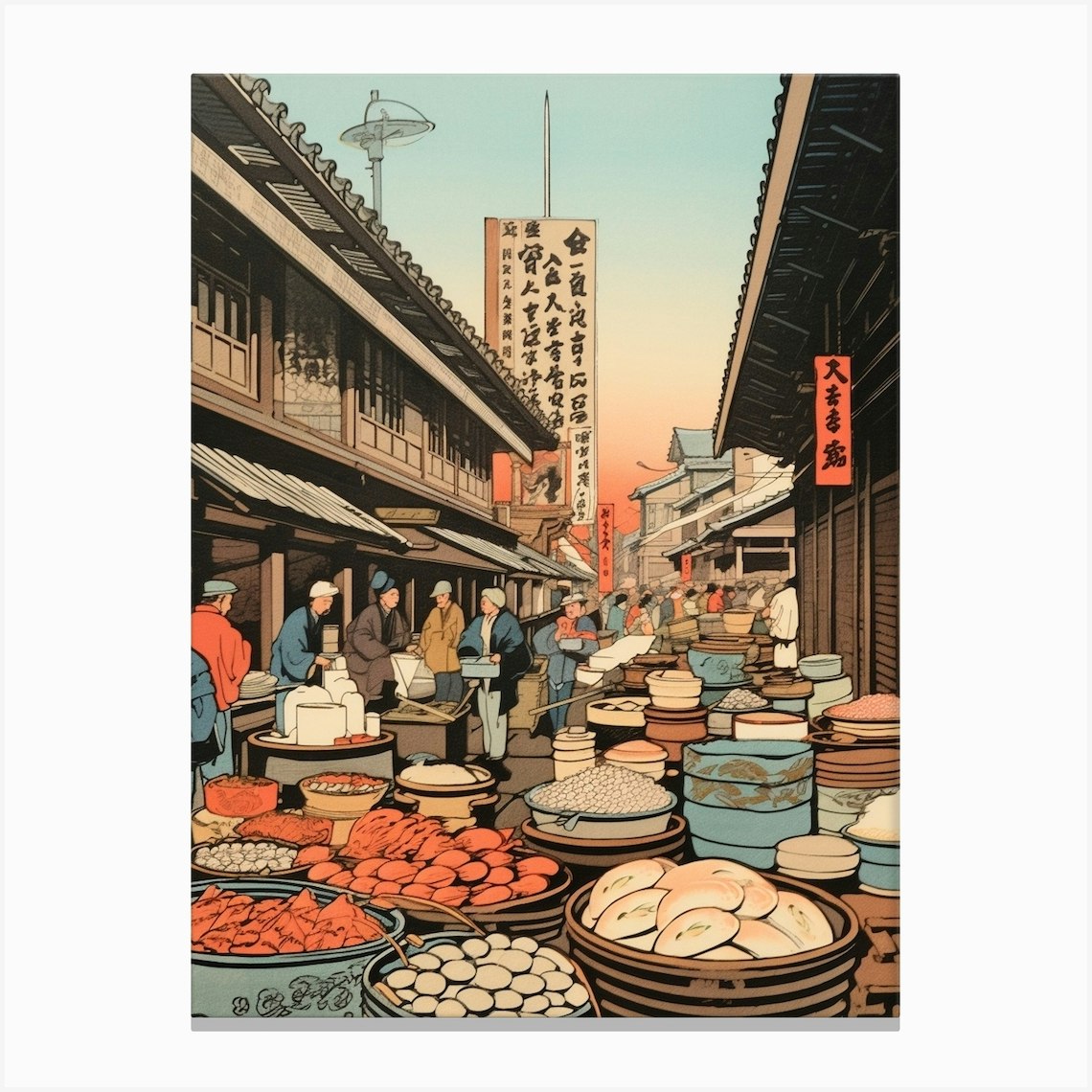The image is a detailed, cartoon-like drawing of a bustling street market set in an old-fashioned Asian town, most likely Japan, based on the signage in Japanese characters. The scene takes place along a narrow pedestrian walkway covered with gray square tiles. On both sides of the street stand traditional buildings adorned with large blue or green tiled roofs. The sky is clear and blue, gradually transitioning to an orange hue near the horizon.

Vendors line the street, their stalls brimming with a variety of goods. These include baskets and containers overflowing with round breads, eggs, lobsters, rice, and other food items. Additionally, there are pottery items prominently displayed. The market is alive with numerous people, both vendors and customers, contributing to the lively atmosphere. Toward the back and middle left of the image, more signage in Japanese can be seen. The drawing captures the essence and vibrancy of a historical outdoor market scene.